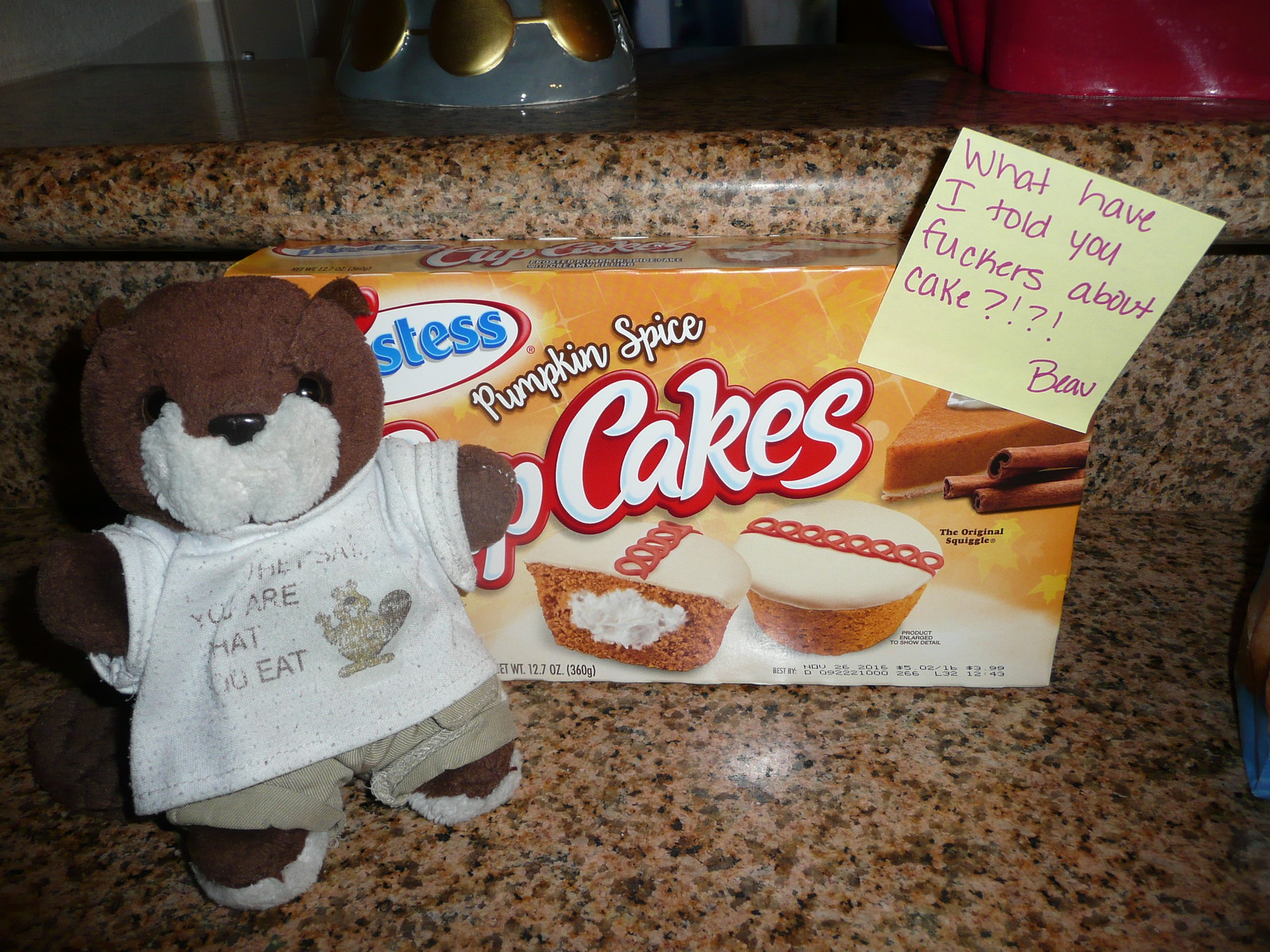In the image, a small stuffed beaver is positioned on the left side of a grainy, marbled, light brown countertop in a kitchen setting. The beaver is wearing faded khaki pants and a t-shirt that says "You are what you eat," featuring a little picture of a beaver. Behind it, there's a Hostess box of pumpkin spice cupcakes, depicting two cupcakes—one cut open to reveal the cream inside—and images of pumpkin pie and cinnamon. At the upper right corner of the box, a pink post-it note is attached, bearing the handwritten message, "What have I told you fuckers about cake?!" followed by Beave's signature. The counter includes a ledge at the back where a couple of coffee mugs or other vessels can be seen, and the room appears to have low lighting. The overall scene seems playful, likely meant as a humorous setup. The prominent colors in the image include shades of brown, white, black, pumpkin spice orange, cinnamon, red, gold, dark gray, and blue.